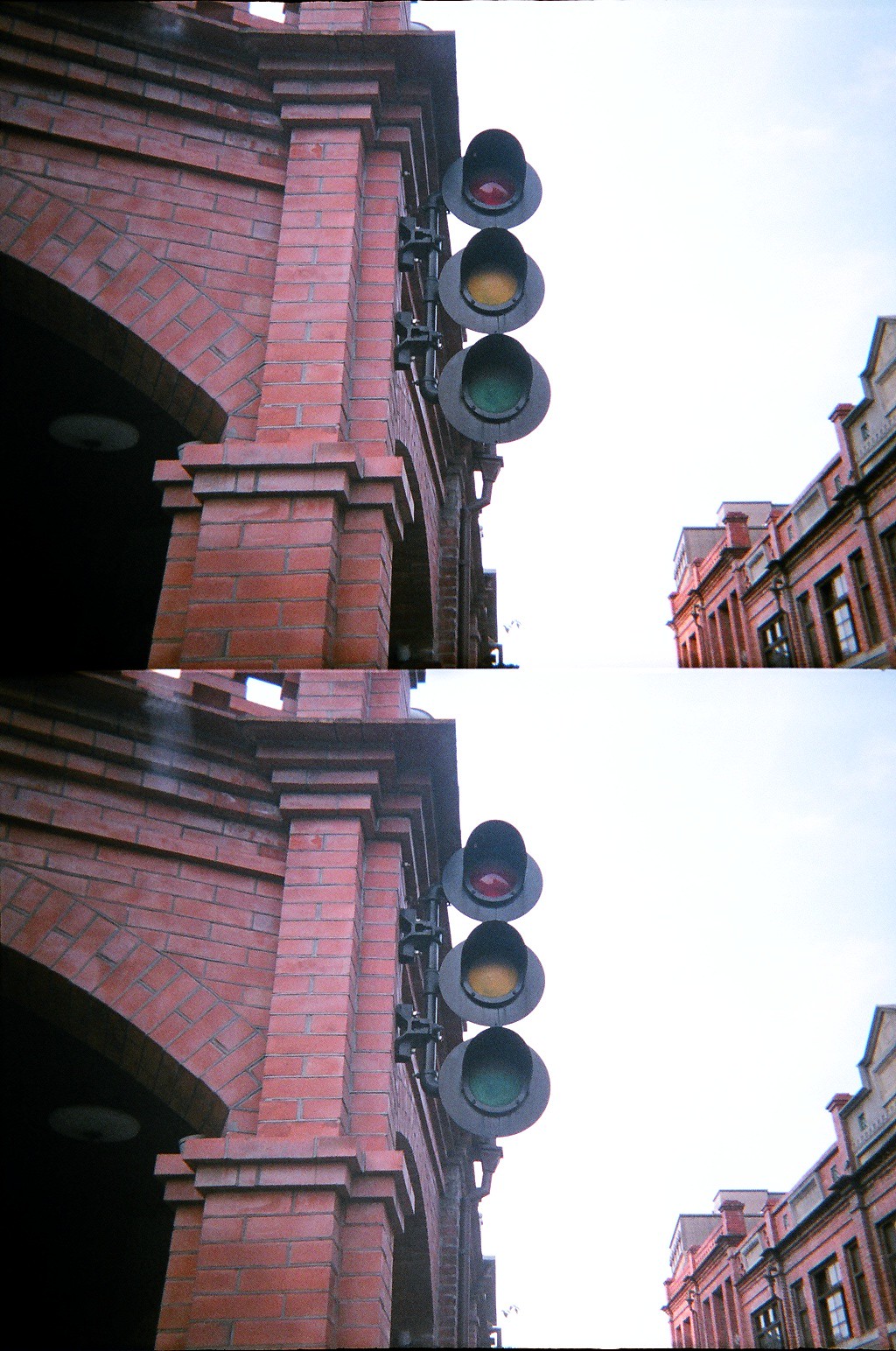This image showcases two nearly identical photographs stacked upon each other, both capturing an old-fashioned traffic light affixed to a red brick building with intricate architectural details. The traffic light, featuring round black housing with red, yellow, and green lenses, is mounted on a black metal structure that curls over the top. None of the lights are illuminated, suggesting the light is inactive or decorative. The red brick building to which the light is attached displays graceful curves just below the attachment point. Both photos also depict another red brick building with windows, a chimney top, and a gray archway visible to the right and in the bottom right corner of the images. The background features a pale, cloudy sky, providing a soft contrast to the rich textures of the brick buildings.